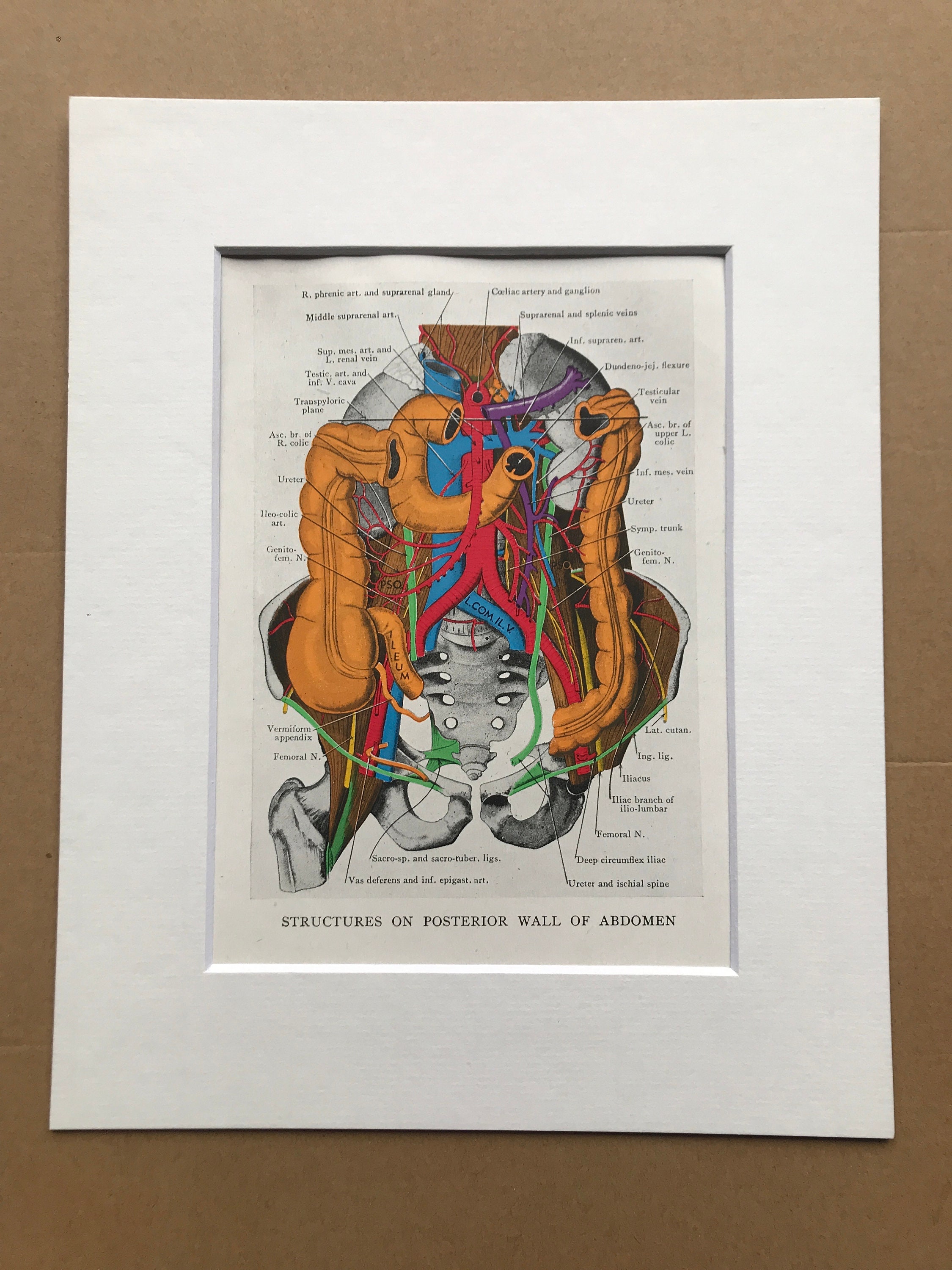The image features a photograph of a framed, detailed colored illustration of human anatomy, specifically labeled "Structures on Posterior Wall of Abdomen." The diagram is set in a wide white matte frame that appears to be made of cardboard. Inside this frame, a printed diagram vividly displays various anatomical components in different colors. The illustration includes prominent parts such as the hip bone in the lower left corner, sections of the pelvis, the large intestines colored in orange, and clearly delineated red arteries and blue veins. Additional structures like the right phrenic artery, suprarenal gland, celiac artery, spleen, and other veins and arteries are labeled in black lettering, with lines pointing to each respective part. While some labels are hard to read due to their size, they comprehensively cover the anatomy of the posterior abdominal wall, making it both an informative and visually engaging depiction.